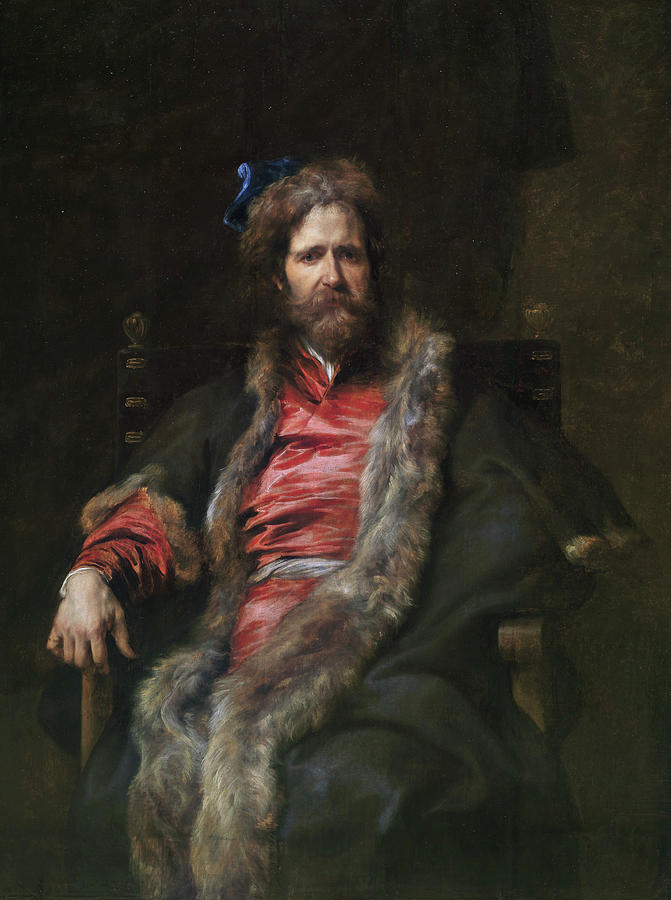The image is a meticulously detailed painting of a man seated in a dark brown wooden chair. The atmosphere of the painting is somber, with a predominantly dark brown and black background that transitions from darker shades on the left to lighter browns on the right. The man, depicted with white skin, sports a fluffy brown head of hair, alongside a bushy brown beard and mustache. Perched on his head is a small blue hat, reminiscent of an Italian cap. His gaze is directed straight at the viewer, adding intensity to his presence.

He is garbed in a layered outfit, starting with a red shirt cinched by a gray belt. Over this attire, he wears an expansive, dark brown fur coat with light brown or cream-colored fur trim that extends from the neckline all the way to the ground, giving the impression of both grandeur and functionality akin to a winter coat. This fur trim is most notably ample around the collar.

In terms of physical presence, his right hand is visible, clasping the chair's side, while his left hand is concealed, possibly bent behind or obscured by his side. The overall effect of the detailed attire and the deep, muted color palette evokes a sense of historical gravity, comparable to figures like a Russian Tsar or an Italian revolutionary such as Giuseppe Garibaldi, though not overly ornate.